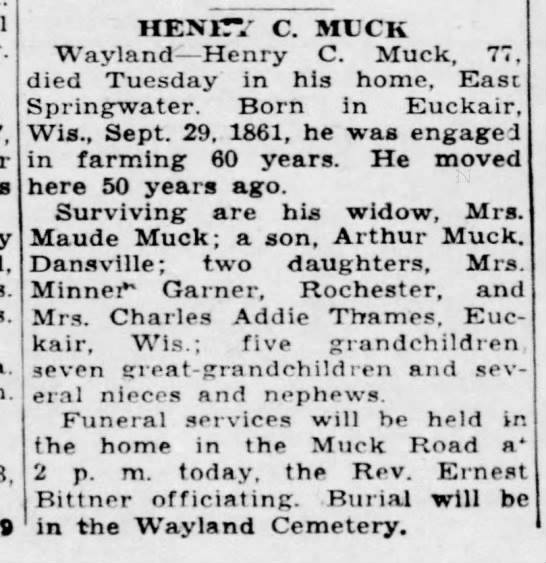This image features an old newspaper obituary that has been cut out and saved. The clipping has a white background with black text, presenting varying levels of clarity; the upper section is darker and bolder, while the lower section appears lighter and somewhat faded against the grayish background. The obituary is bordered by black bars on both sides, separating it from adjacent articles, with some partial letters from another advertisement on the left.

At the top, prominently displayed in dark black text, is the name "Henry C. Muck". Below this, a slightly less bold but still readable description follows detailing the life and death of Henry C. Muck, from Wayland, who died at age 77 on a Tuesday in his home in East Springwater. He was born on September 29, 1861, in Ucare (or possibly Ockair), Wisconsin, and spent 60 years engaged in farming. He moved to his final residence 50 years prior to his passing.

The obituary lists his surviving loved ones: his widow, Mrs. Maude Muck; a son, Arthur Muck from Dansville; and two daughters, Mrs. Minna Garner from Rochester and Mrs. Charles Addy from Thames. Additionally, he is survived by five grandchildren, seven great-grandchildren, and several nieces and nephews. The funeral services are slated to be held in the home on Muck Road at 2 p.m., officiated by Reverend Ernest Bitter, with burial to take place in the Wayland Cemetery.